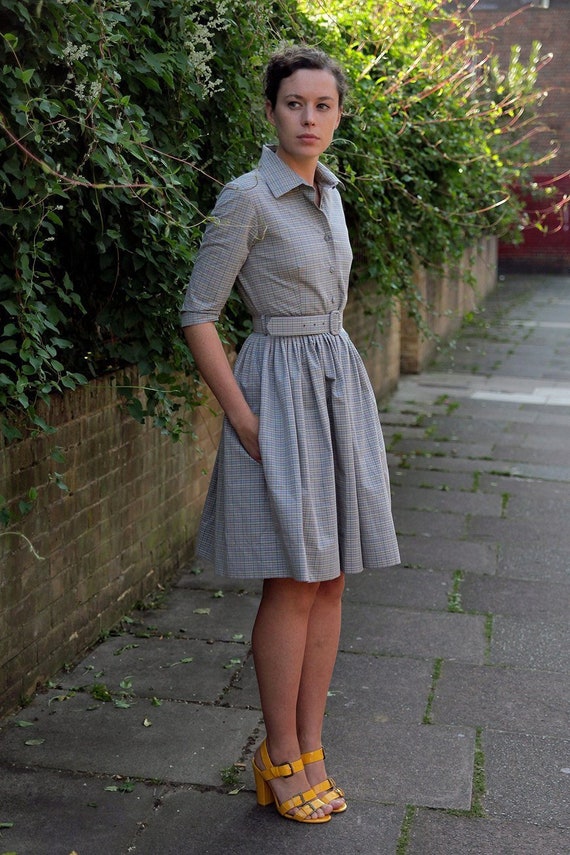A young white woman, appearing to be in her early 20s, stands on a cement sidewalk with little bits of moss growing between the stones. She has brown hair pulled back and is dressed in a light blue, plaid-patterned outfit consisting of a matching top and skirt that extends to her knees. The top has elbow-length sleeves and a shirt collar, buttoning down to the waist, which is cinched with a matching belt featuring a buckle at the front. She is wearing high-heeled, yellow strappy sandals. She is positioned slightly angled to her right, but her face is turned toward the left, gazing away from the camera. Behind her, a dirty brown brick wall about waist-high supports thick, dark green shrubs with a few small white flowers interspersed. The sunlight illuminates the foliage behind her, creating a stark contrast with the stone pathway she stands on.